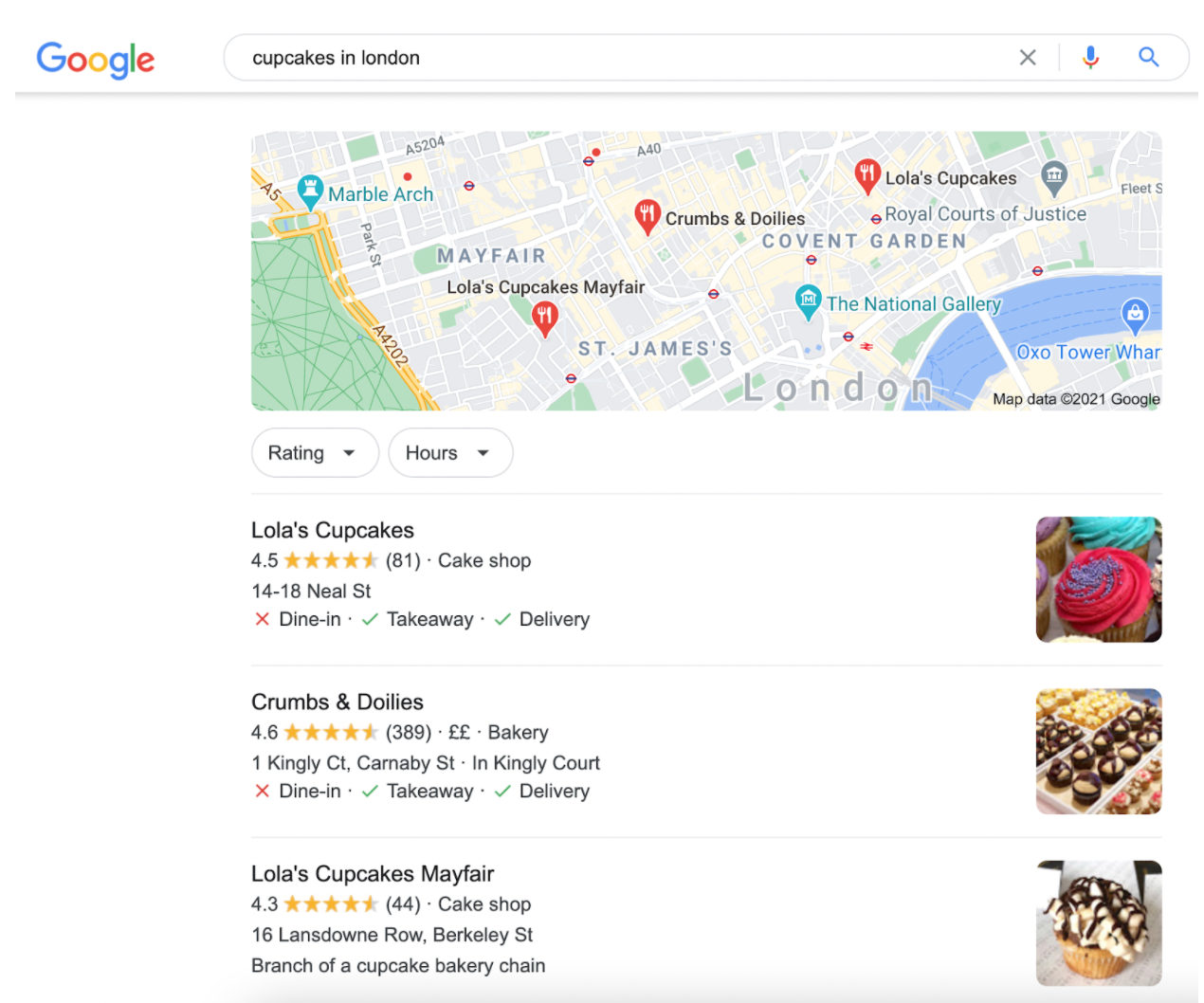The image depicts a Google search results page for "cupcakes in London." The iconic Google logo is prominently displayed at the top left in its traditional blue, red, yellow, and green colors. Directly to the right is the search bar with the query "cupcakes in London" entered. Within the search area, there is an 'X' symbol on the far right, followed by a vertical line, a microphone icon, and a magnifying glass icon indicative of the search function.

Beneath the search bar, there appears to be a map section populated with various location markers. Three of these markers are orange and feature a fork and knife symbol, signifying places to eat. Other markers depict icons such as buildings and shopping carts or purses, indicating different types of establishments.

Further down, there is a section for filtering the results with options for "Ratings" and "Hours," each accompanied by a drop-down arrow for additional selections. This is followed by three rows representing individual listings of cupcake shops.

The first listing is for "Lobos Cupcakes," which boasts a rating of 4.5 stars. It identifies itself as a cake shop and provides the address. Icons indicate available services: dine-in (marked with an 'X'), take away (checked), and delivery (also checked). To the right of this listing, there are images of the cupcakes.

The same format is used for the other two entries: "Crumbs and Doilies" and "Lola's Cupcakes Mayfair." Each listing includes the shop's name, ratings, type of establishment, address, service options, and corresponding images.